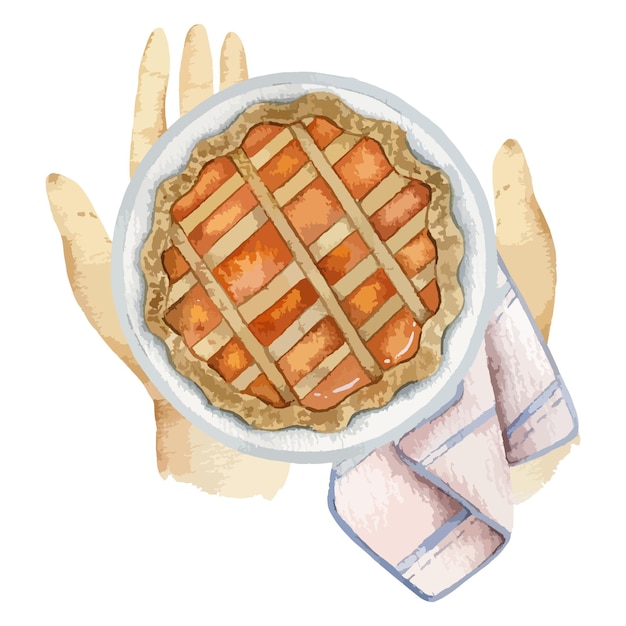This is an illustration, likely done in watercolor, depicting two Caucasian hands with detailed lines, holding a small, well-baked pie. The hands are using a folded, pinkish-white dish cloth with blue stripes to help grip the pie dish, which is light gray. The pie features a light tan crust with wavy, crimped edges and a lattice pattern that is slightly irregular, exposing a vibrant orange filling beneath it. The dish rag and the pie dish share similar colors, adding to the cohesive style of the artwork. The pie, possibly peach or apple, rests in a pie dish centered between the hands and occupies about half of the left hand’s surface.